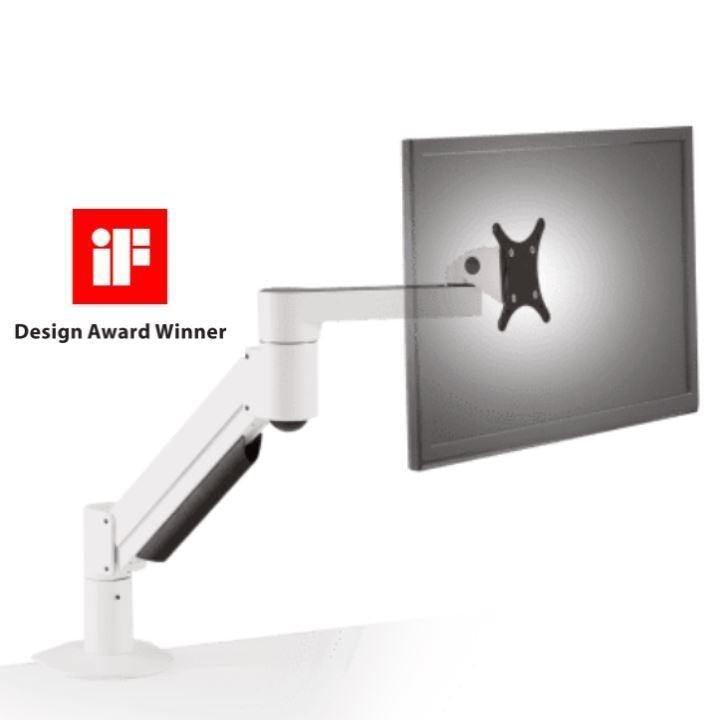This image depicts a sophisticated monitor or screen holder that has won an IF Design Award, as indicated by a red square with "IF" and black text stating "Design Award Winner" on the left side of the photo. The holder features a large, gray screen attached to a sleek, movable white arm with multiple articulated joints. These joints include a white tube that rises from a circular base, transitioning into a diagonal segment with black lining underneath, and culminating in a black attachment secured by four screws. This arm ensures flexibility, allowing the screen to be adjusted closer or repositioned easily. The base of the arm includes a distinct black ball component, further adding to its maneuverability. The intricate design suggests this stand could support a television or computer screen, offering both functionality and award-winning design aesthetics.